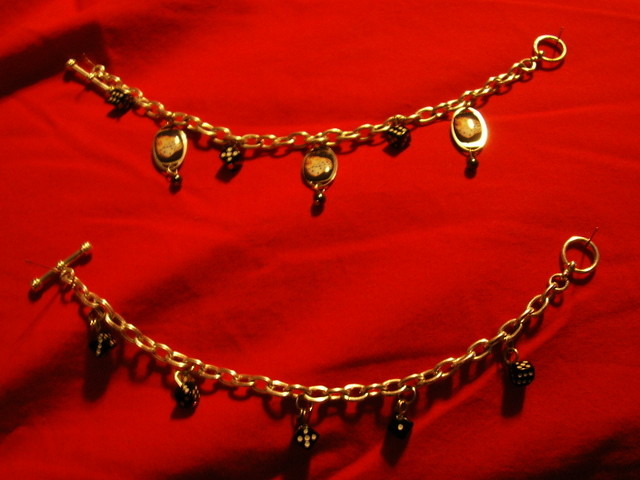This color photograph showcases two intricately designed gold chain bracelets adorned with small charms and trinkets, spread out flat on a slightly wrinkled red linen tablecloth. The bracelets, positioned one above the other, occupy nearly the entire width of the image. The red cloth beneath them features creases and waves, particularly noticeable towards the upper left and bottom edges, creating dark shadows that accentuate the fabric's texture.

The bracelets are arranged in an upward-facing oval shape and are not closed, with each having a clasp mechanism—the circular end on the right and the 'T-bar' end on the left for securing. The upper bracelet displays several roundish charms that are more visible, featuring both gold and black accents. The lower bracelet, partly obscured by shadows, also has similar decorative elements, including a cross and what seem to be dice charms adorned with visible numbers and dots like five, two fives, one, and possibly a six. Some charms on the upper bracelet also resemble tags with images of dice, each depicting three dice. The detailed craftsmanship and arrangement on the vivid red cloth make the jewelry stand out beautifully in the photograph.